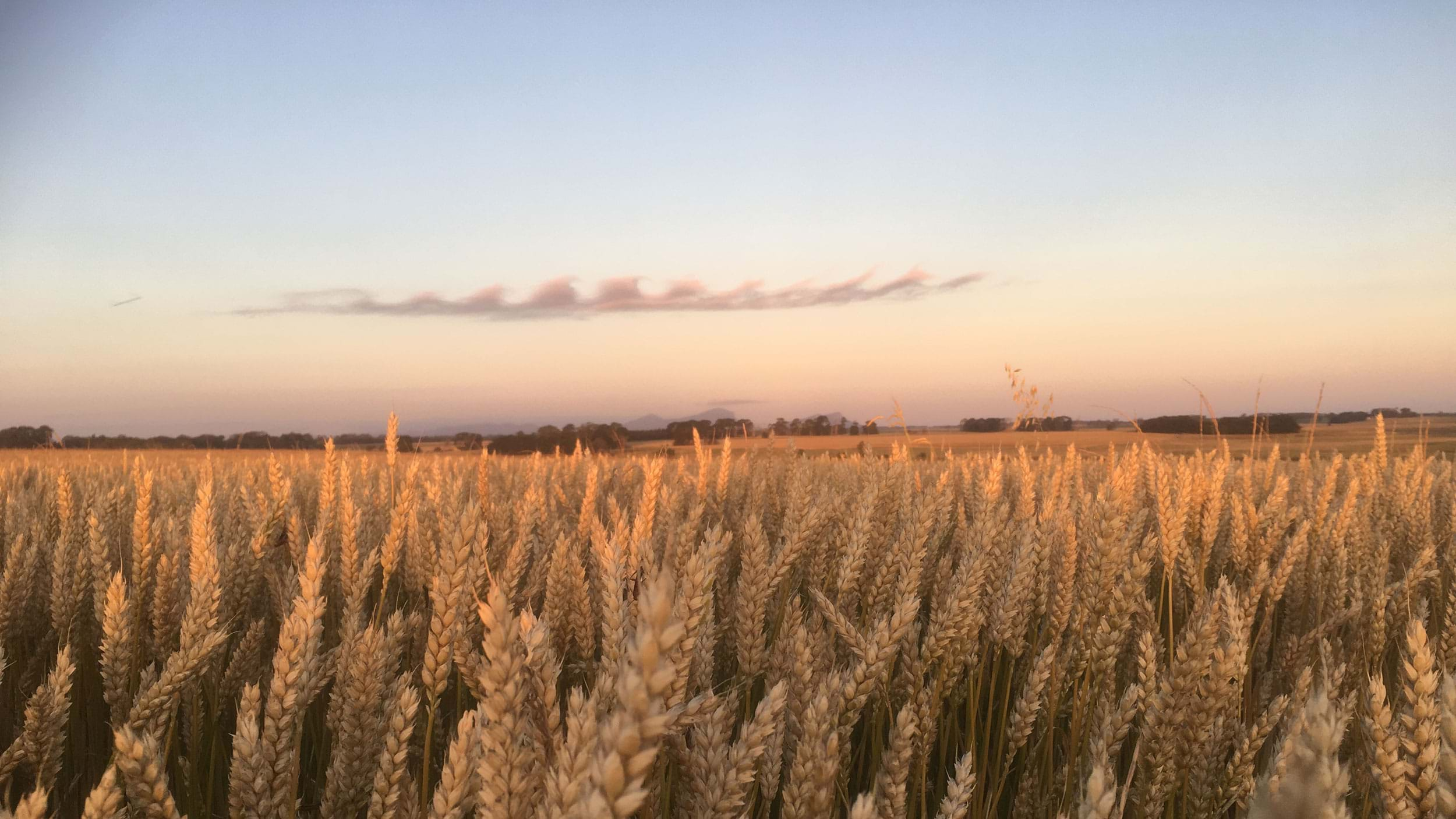The image captures a vast, open field of golden wheat that stretches to the horizon under a clear sky. The wheat stalks stand tall, swaying in the wind, giving a sense of movement and vitality to the scene. The sky above transitions from a soft pinkish-yellow at the bottom to a tranquil blue at the top, suggestive of a sunset or dusk setting. A snake-like, wispy cloud drifts through the middle of the sky, adding to the serene atmosphere. Distant trees and what appear to be barns dot the horizon, grounding the scene within an agricultural or farm setting. The photograph is rich in color, featuring the soft pastels of the sky and the warm tones of the wheat, creating a picturesque and peaceful rural landscape.